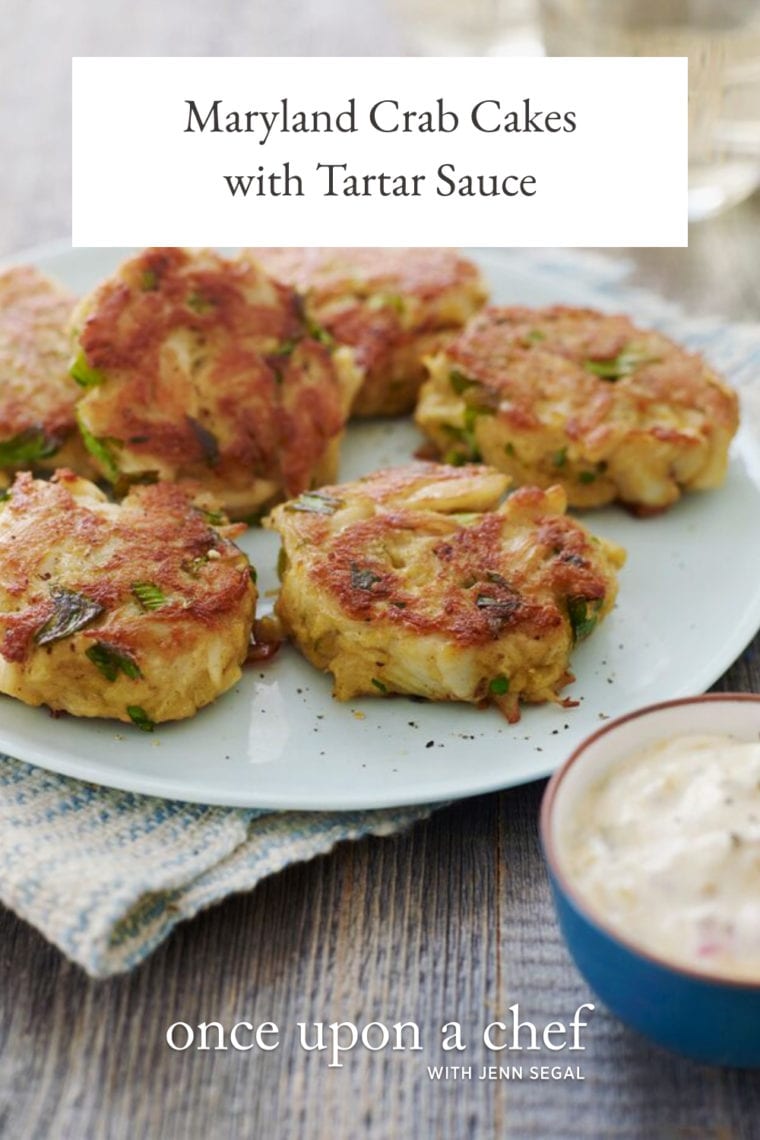The image is a detailed photograph of six golden-brown Maryland crab cakes, arranged on a white plate. The crab cakes have a crispy, fried exterior and are speckled with hints of yellow, white, and green from scallions mixed into them. One crab cake is slightly propped up on the upper left side of the plate. The plate itself rests on a kitchen towel, which in turn lies on a wooden table. In the lower right corner of the image, there is a small blue ramekin with a brown rim, filled with creamy white tartar sauce. At the top of the image, a white rectangle contains black text that reads "Maryland crab cakes with tartar sauce." At the bottom of the image, also in white letters, appears the text "Once Upon a Chef with Jen Seagal."